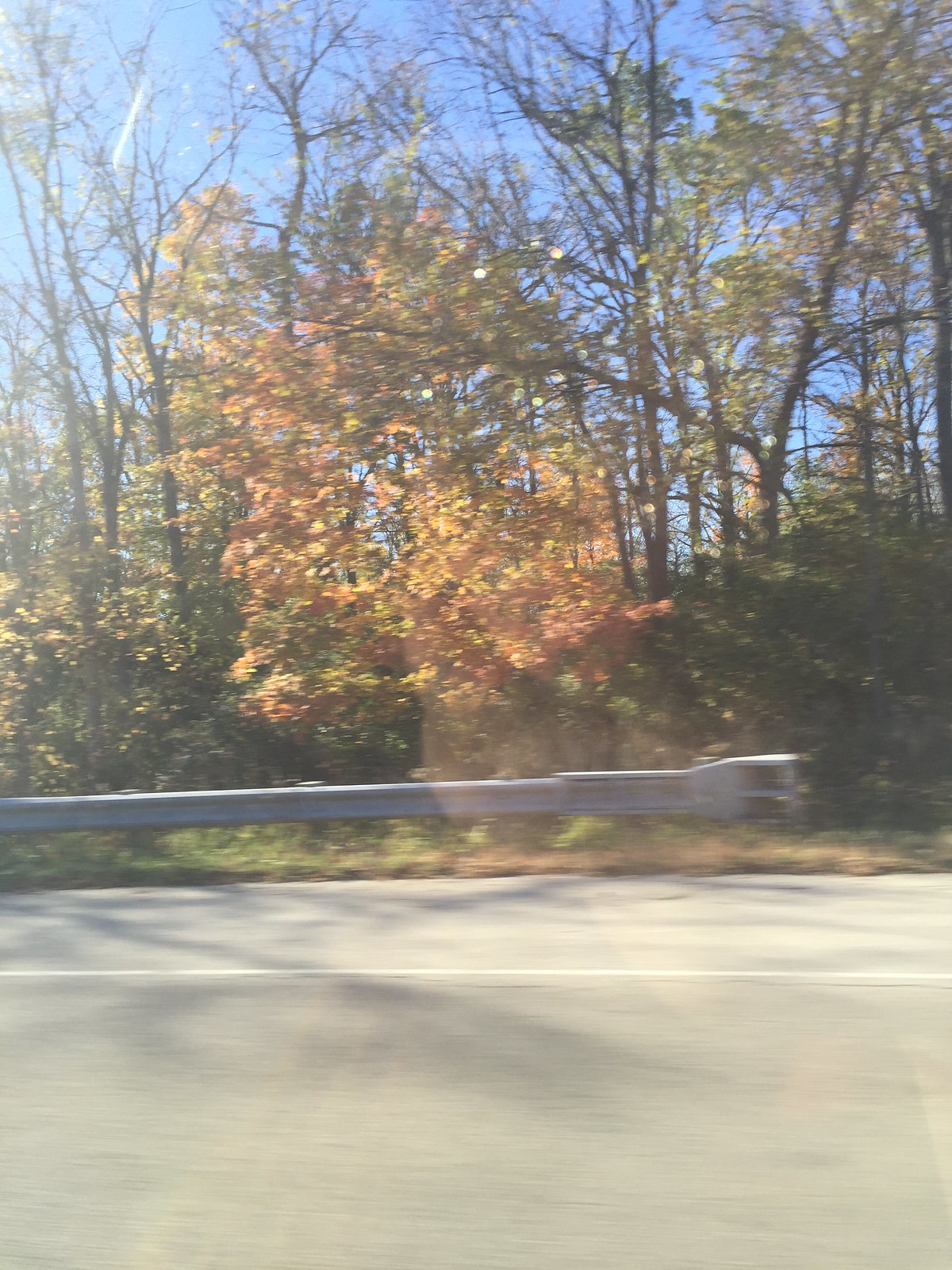This photograph, seemingly taken through a vehicle window, captures a roadside scene that is slightly blurred, likely due to the moving vehicle. The sky overhead is an unblemished bright blue, contrasting sharply with the bare trees that populate the scene, devoid of leaves. However, a section of the image reveals a tall bush still clinging to its autumn colors, with yellow and scattered orange leaves. In the foreground, a few green bushes add a splash of color to the otherwise muted landscape. The bottom of the image features a silver guardrail running parallel to the road, demarcating the roadside from the asphalt. A narrow, auxiliary lane borders the main road, distinguished by a pale gray hue and a white line separating the two paths. The combined elements create a vivid snapshot of a transitional season viewed from a moving car.